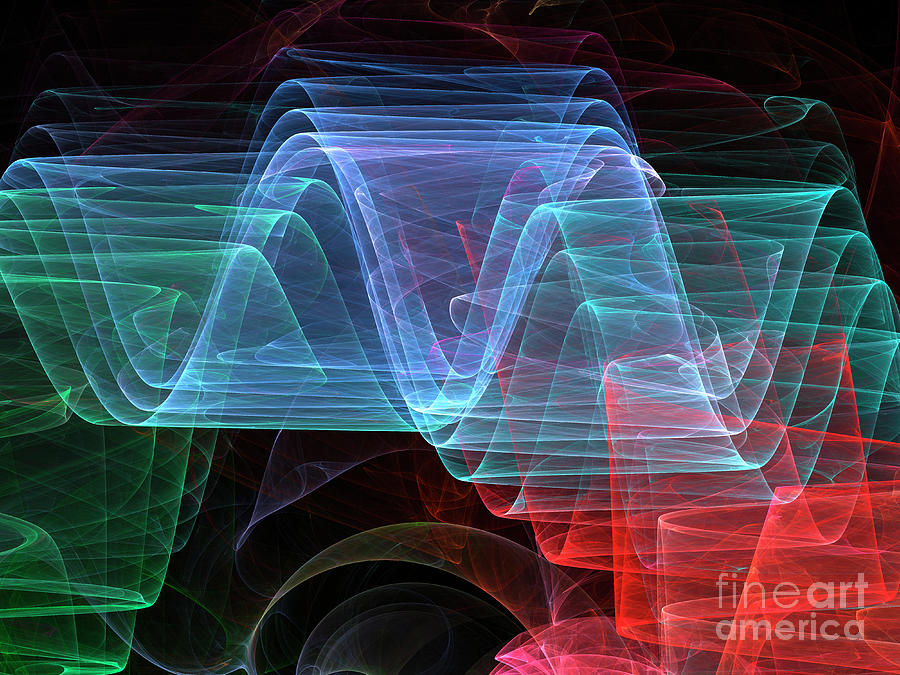This digital artwork, presented on a computer-generated medium, showcases a mesmerizing semi-abstract composition. Set against a stark black background, the image features a series of undulating waves crafted with precision using digital tools. These waves ripple across the canvas in a visually captivating pattern, with each iteration of the wave exhibiting subtle variations in color. The palette includes shades of blue, aqua, green, red, and purple, creating a vibrant contrast against the dark backdrop. The harmonious blend and repetition of these colors generate a dynamic sense of movement and depth. In the bottom right corner, a watermark from Fine Art America serves as a signatory element, affirming the authenticity and source of this captivating piece.